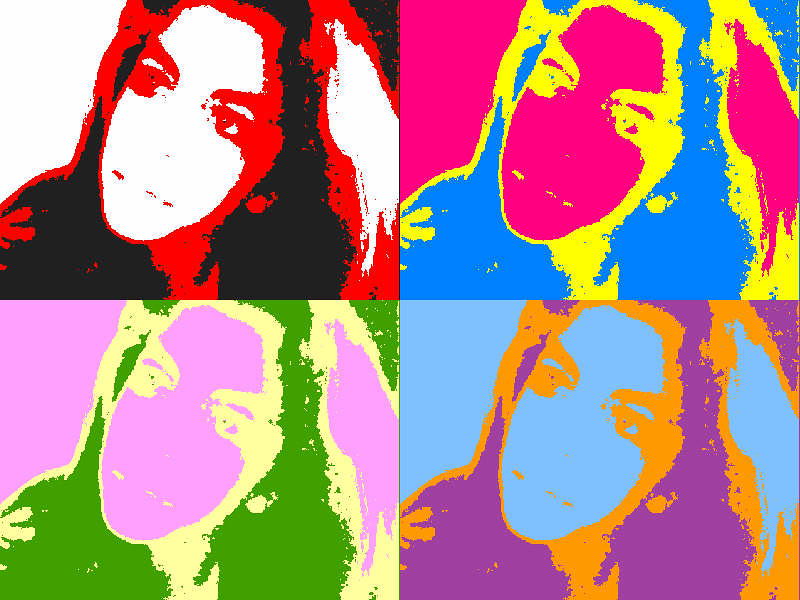The image features a pop art collage divided into four equal squares, each depicting an overexposed illustration of a woman with long dark hair gazing towards the upper left corner. The woman’s head is tilted to the right and she has distinctively detailed eyes, lips, and nostrils, adding depth to the stylized representation. Each quadrant varies in vibrant color schemes:

- **Top Left Quadrant:** The woman's face is white, with red accents on her lips and nostril. Her hair and clothing are rendered in black, contrasted against a red background.
  
- **Top Right Quadrant:** The woman's face, hand, and top left corner are neon pink. Her eyebrows, eyes, nostril, and lips are neon yellow, while her hair and clothing are depicted in neon blue.
  
- **Bottom Left Quadrant:** The face and hands of the woman are a light lavender purple. Her facial details and the aura around her hand are a yellowish off-white, and her hair and outfit are bright green.
  
- **Bottom Right Quadrant:** Here, her face and hands are light blue, with the facial features and hand aura in orange. Her hair and body are presented in a deep purple.

Each section harmoniously combines diverse hues to create a captivating and dynamic visual effect reflective of the pop art style.